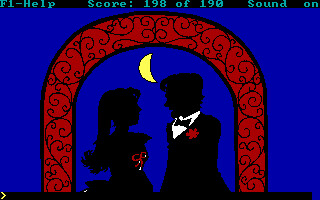The image appears to be a scene from a 1990s video game, depicting a wedding. The screen is framed by narrow black borders at the top and bottom. Within the bottom border, there's a small yellow arrow resembling a right-pointing "V," similar to an arrow key on a keyboard. The upper border features several pieces of information in light blue text: "F1-Help" is displayed on the far left, followed by "Score: 198 of 190" slightly to the right, and "Sound ON" further towards the right.

The main image has a blue background and is dominated by a red arch with a black decorative pattern running through it. In the center of the scene, the silhouetted figures of a bride and groom stand beneath the arch. The bride, positioned on the left, wears a dress adorned with a red bow. The groom, on the right, is dressed in a classic black tuxedo with a white undershirt, a black tie, and a red flower pinned to his lapel. A yellow crescent moon is positioned between the couple, completing the romantic imagery.